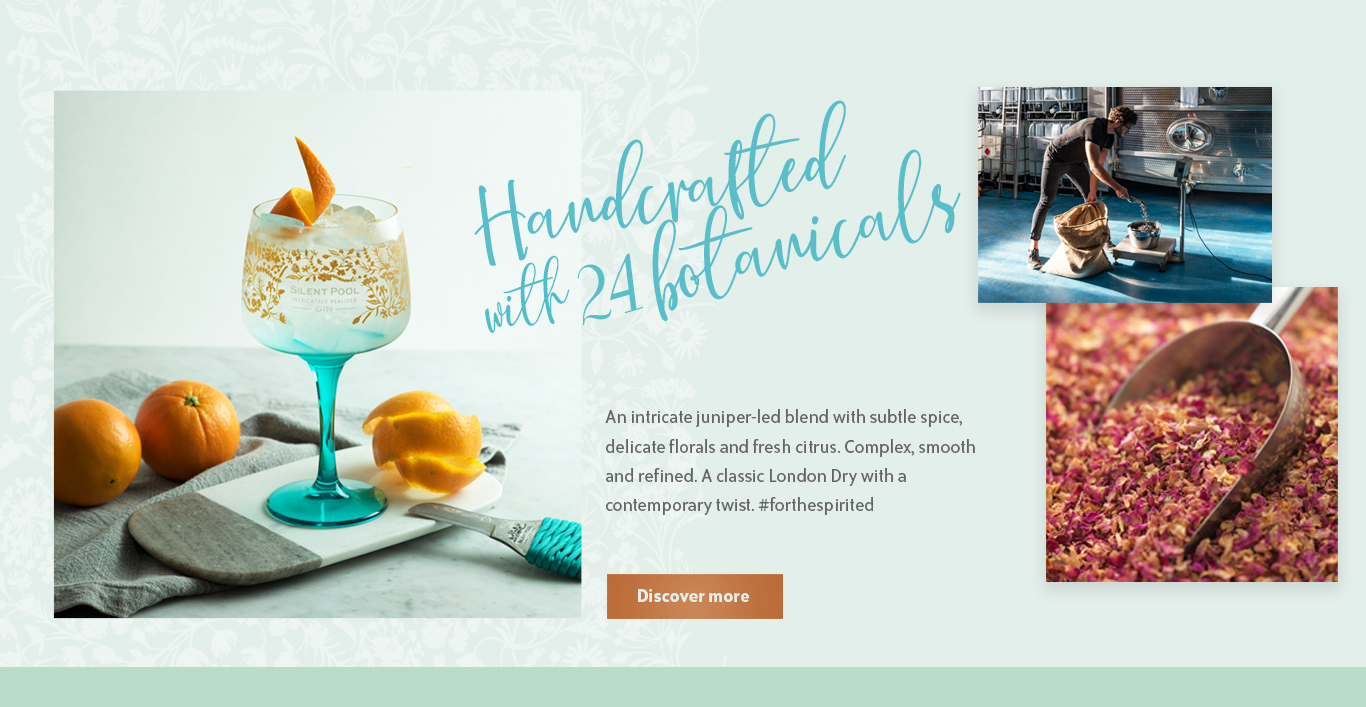The website features a pale blue-grey, stencil-style floral background. On the left, there is a prominent image of a drink in a frosted glass with a teal stem. The glass holds a drink with ice and a garnished orange peel. The drink sits on a non-circular, white rectangular plate with a grey section at one end. Additional curled orange peels and a knife rest on the plate, which is placed on a grey tea towel. Two oranges lie further back on the tea towel, which is set on a whitish-grey countertop. The background wall is a light white.

In the middle of the page, scripted text in a blue font states, "Handcrafted with 24 botanicals." To the right, there is a smaller image of a man pouring something into a bucket over scales, although the details are hard to make out. Below this, another image features dried flowers and a metal scoop.

Below these images to the left, a text block describes the drink: "An intricate juniper-led blend with subtle spice, delicate florals, and fresh citrus. Complex, smooth, and refined, a classic London dry with a contemporary twist. Hash for the spirited." At the bottom-center of the page is a brown button with white text that reads, "Discover More." Finally, a darker blue-green border runs straight across the bottom of the page.